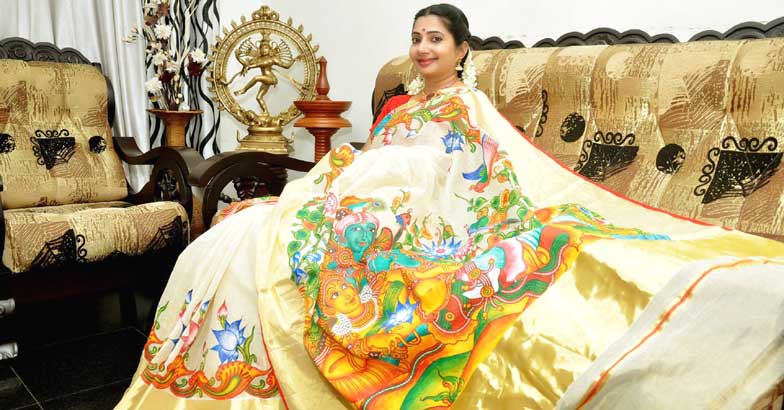In this photorealistic image, a South Asian woman with dark hair, adorned with large dangly white earrings and a bindi, is seated and smiling on a golden couch adorned with black designs toward the right of the image. She is elegantly dressed in traditional South Asian attire—a cream-colored sari or gown enriched with intricate patterns and vivid depictions of Hindu gods and flowers, which cascades toward her right onto the couch. To her left is a matching gold and black upholstered armchair. Between the couch and the armchair sits a side table bearing a gold decorative statue framed in a ring-like structure, suggestive of an Indian deity, and a gold vase with white flowers. The scene is set against a backdrop of white curtains and a white wall, enhancing the sense of elegance and cultural richness.